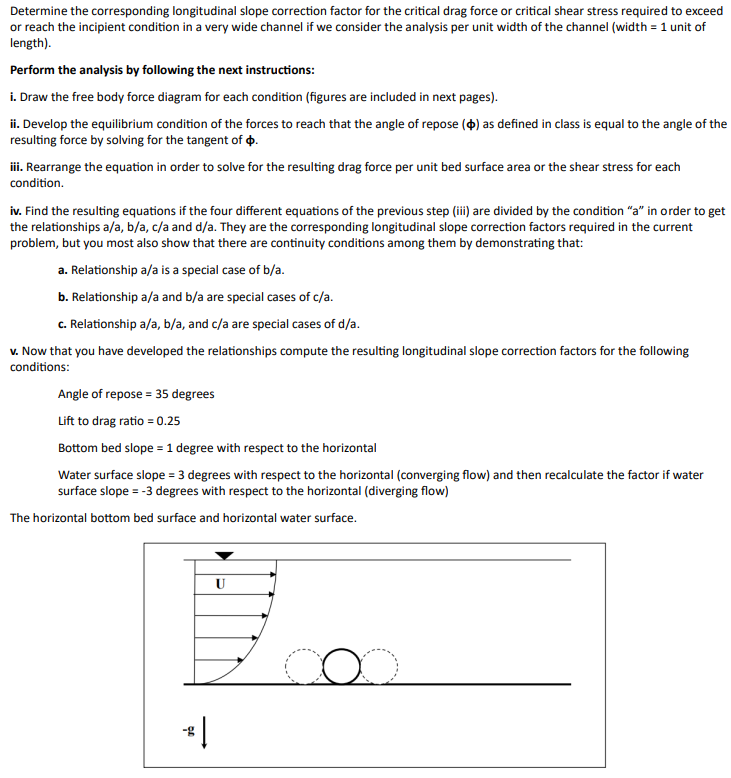The image depicts a highly detailed page from a scientific or engineering textbook, focused on determining the longitudinal slope correction factor required for critical drag force or critical shear stress in a very wide channel. The background is white with black text, and the instructions are numbered. The excerpt instructs on drawing free-body force diagrams, developing the equilibrium conditions, and rearranging equations to solve for drag force or shear stress per unit bed surface area. The text elaborates on calculating longitudinal slope correction factors under specified conditions, such as an angle of repose of 35 degrees, lift-to-drag ratio of 0.25, bottom bed slope of 1 degree, and water surface slopes of 3 degrees and negative 3 degrees.

At the bottom of the page is a diagram featuring a 'U' shape with arrows pointing to the right, representing forces typically seen in a physics context, such as gravity and other forces in action. The diagram includes three circles aligned horizontally, some solid and others with slanted lines, alongside a vertical arrow marked with '-G' indicating gravitational force. The page provides a blend of complex theoretical analysis and visual aids to help understand the dynamics of forces in wide channel flow systems.